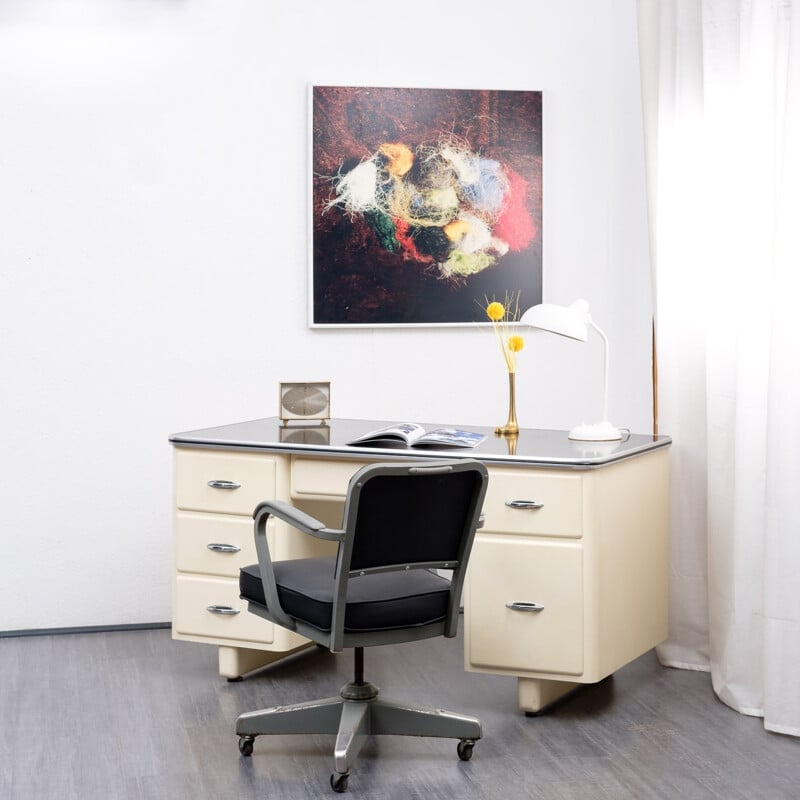This photograph captures a well-organized home office featuring a cream-colored vintage desk with a metallic silver top, chrome handles, and three drawers on the left side, two drawers on the right side, along with a centered drawer partially obscured by an office chair. The chair, with its black fabric seat and steel armrests cushioned with plastic or felt, sits on black wheels facing the desk. The desk hosts an open notebook, a brass clock with a square face and brass components, and a brass vase holding yellow flowers. Adjacent to these items stands a white adjustable table lamp. The office setting is lightened by sunlight streaming through white floor-to-ceiling drapes. A striking feature on the plain white back wall is an abstract painting depicting colorful yarn-like figures with hues of white, orange, beige, green, red, black, and yellow against a brown fading into black background. The room is anchored by beige or gray fake wood flooring, creating a homely yet professional atmosphere.